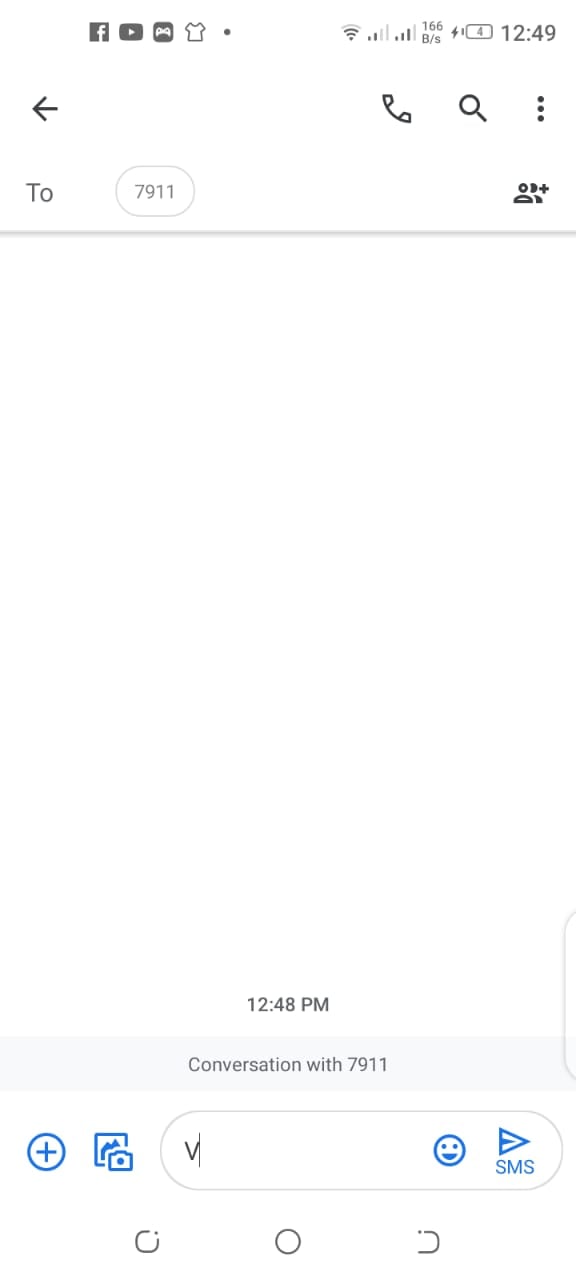A screenshot of a smartphone screen showcasing a minimal yet detailed interface. At the upper section of the screen, there's significant white space, prominently featuring a gray header. On the left of this header, there are icons for Facebook, YouTube, a video game controller, and a t-shirt, while the right side displays a Wi-Fi icon, two signal strength indicators (one with two bars, the other with three, out of a maximum of four), followed by "166B-S," a lightning bolt, a battery icon with a '4' (indicating unknown metrics, possibly four hours or four percent), and a clock showing 12:49.

Below this, a navigation bar includes a back arrow on the left and three icons on the right: a phone receiver, a magnifying glass, and a menu (denoted by three dots). Underneath, there is the number "2" displayed next to "7911," encapsulated in a thin-lined gray capsule shape. To the right, there are two stacked profile icons with a plus sign beside them.

The middle portion of the screen is mostly empty white space, offering a clean and uncluttered design. At the bottom, the screen displays "12:48 p.m.," indicating the time of a conversation with "7911." Further elements on this lower section include a plus sign within a circle, a photo icon with a camera overlay, a search bar with the text "V" and a blinking cursor, an emoji icon, and an airplane icon labeled "SMS," along with the essential navigation menu at the very bottom.